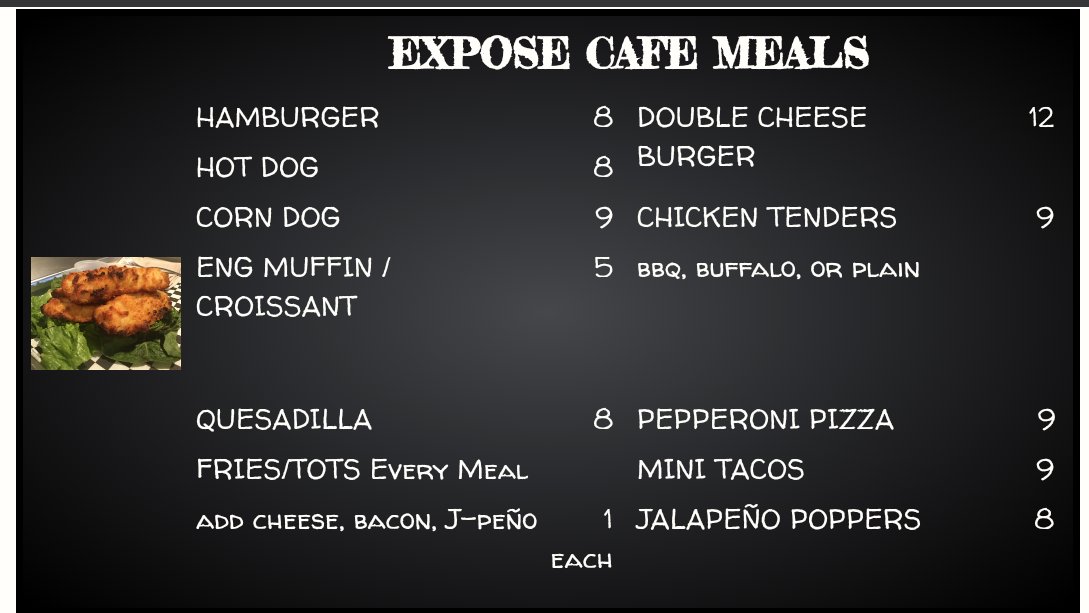In the image, the text "EXPOSÉ CAFÉ MILLS" is prominently displayed in uppercase white letters against a black background at the top. On the left side of the image, there are green lettuce leaves with a couple of pieces of chicken neatly placed on top. 

Starting from the left, a detailed menu is listed as follows:

- Hamburger
- Hot dog
- Corn dog
- ENG muffin/croissant
- Quesadilla
- Fries/tots with every meal
- Add cheese, bacon, J-pinot

Following these items, there is a vertical column of numbers: 8, 8, 9, 5, 8, 1. 

On the right side of the image, additional menu items are listed:

- Double cheese with the number 12 next to it, and the word "burger" underneath
- Chicken tenders with the number 9 to the right, followed by the options "Barbecue, Buffalo, or Plain"
- Pepperoni pizza with the number 9 beside it
- Mini tacos with the number 9 beside it
- Jalapeno poppers with the number 8 about an inch and a half to the right

At the bottom of this menu section, the word "each" is displayed.